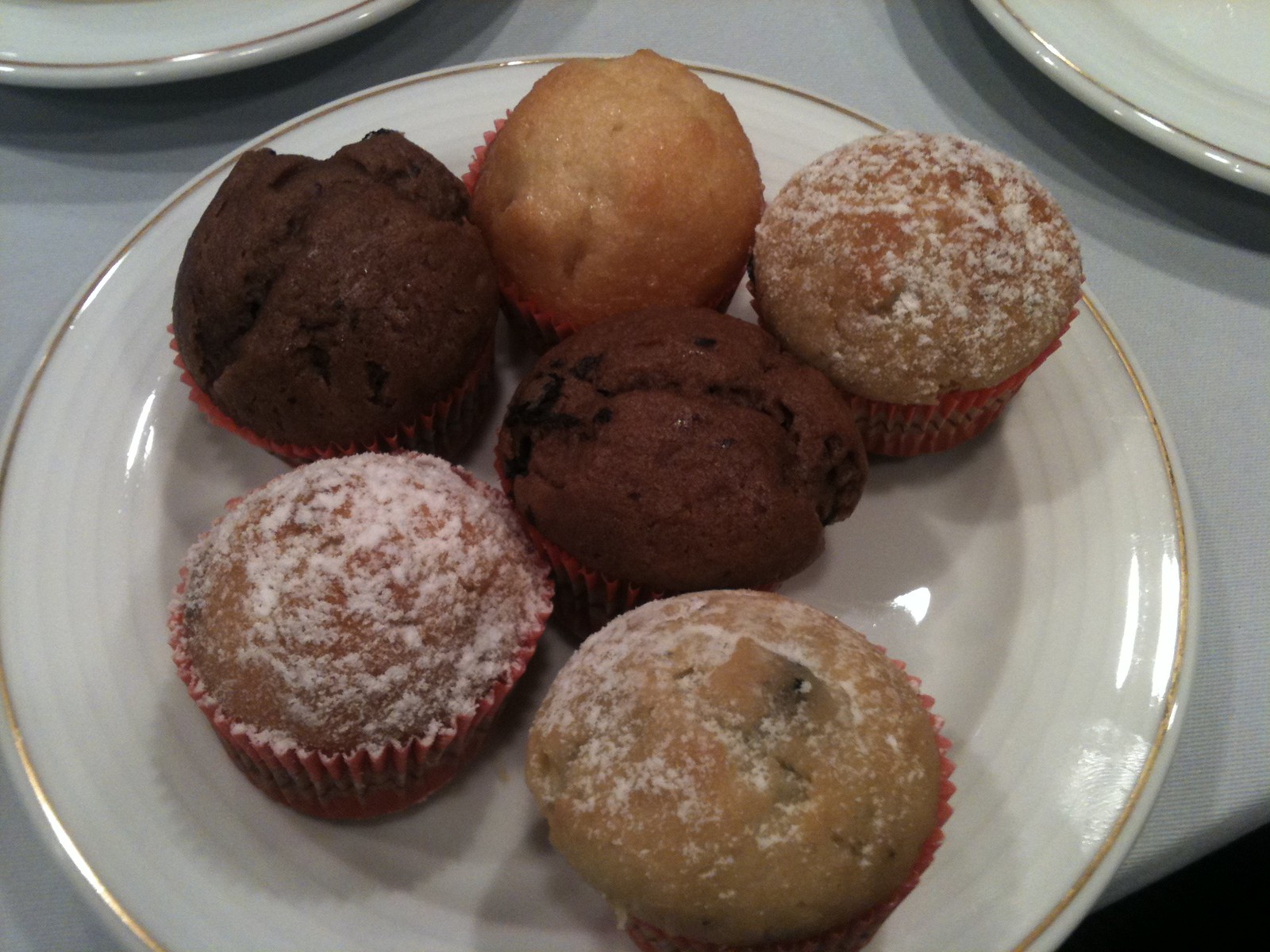The image features a close-up of a table covered with a white or light gray tablecloth. At the center of the table is a plate, more akin to a large saucer, distinguished by a gold band around its edges and decorative circles. This plate, partly obscured at the bottom, hosts six muffins in red paper wrappers. The muffins include two with powdered sugar topping, two that appear to be chocolate, one that is most likely a blueberry muffin with visible blueberries and sprinkled sugar, and another one without any visible toppings or fruit, possibly plain or vanilla. Only portions of two other similarly styled plates are visible in the upper left and upper right corners of the image, adding depth and context to the scene.